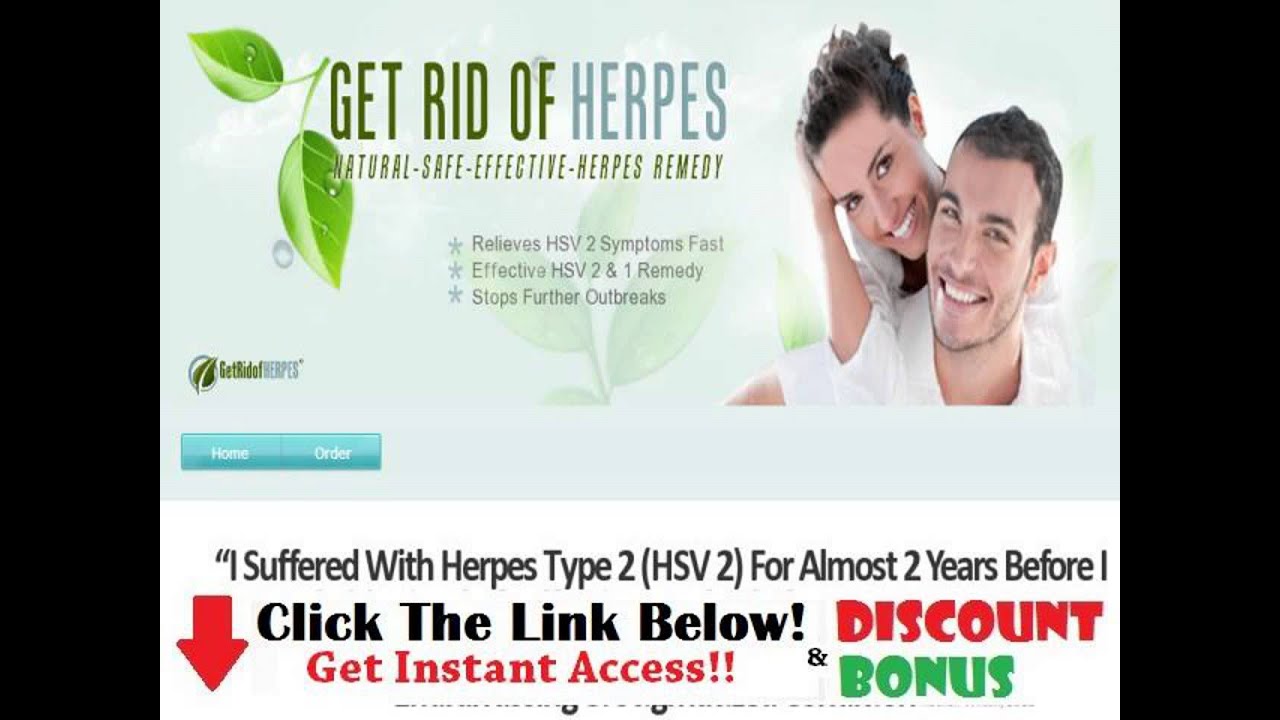This image is a screenshot from an online advertisement for a natural, safe, and effective herpes remedy. The ad prominently features two green leaves at the top, adorned with glistening water droplets. On the right side of the image, a man and woman are pictured close together; the man's in the forefront, while the woman's arm is draped over his shoulder, bringing their faces near each other.

In the center of the image are three gray stars with text underneath proclaiming, "Relieves HSV-2 symptoms fast." Additional text in the middle reads, "Effective HSV-1 and HSV-2 remedy," followed by the claim, "Stops further outbreaks." 

Below, a teal-colored banner includes the options "Home" and "Order." In black print, a testimonial states, "I suffered with herpes type 2 (HSV-2) for almost two years before I...," suggesting action by clicking a link below which offers "Get instant access." A prominently displayed red arrow points downward towards this link.

At the bottom of the ad, key phrases highlight the offer: "Discount" in red, "Bonuses" in green, and "Get instant access" in red.